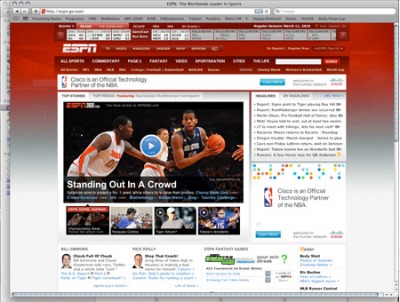The image depicts an ESPN sports webpage viewed from a distance, causing much of the text to appear blurred. Dominating the scene is a main article or video titled "Standing Out in a Crowd," marked by a prominent blue circular button with an arrow, indicating that clicking it will play a video. At the top of the webpage, there's a section displaying various sports scores and categories for different sports that users can click on. In the bottom left and slightly middle left areas of the screen, images of two writers are visible; clicking on their images or the accompanying text will open their articles. On the right side of the webpage, the NBA logo is displayed with the text "Cisco is an official technology partner of the NBA." This message also appears above the main video, reinforcing Cisco's partnership with the NBA.